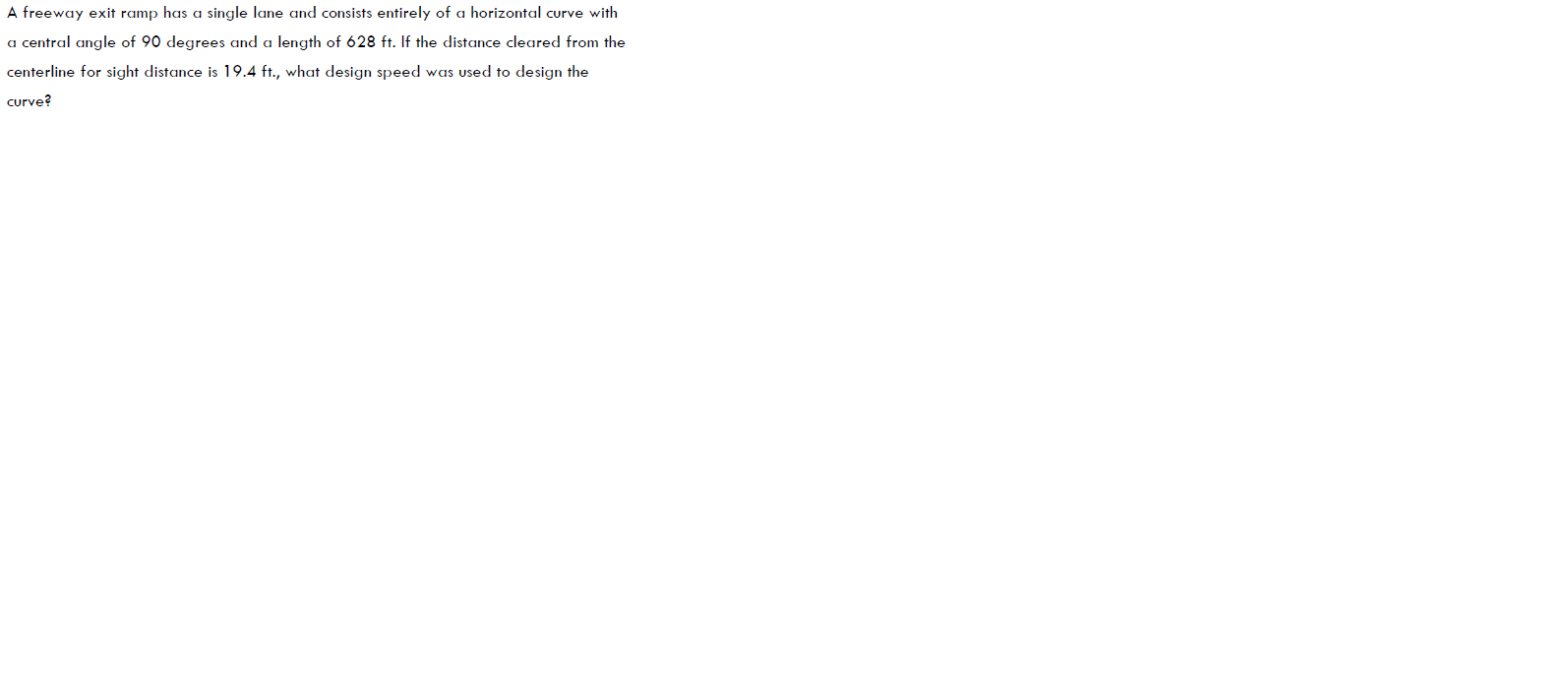This is an image of a screenshot displaying a portion of text against a white background. The text appears in the upper left corner, suggesting that additional content is intended to appear on the screen but is currently missing. The text is presented in a very small, dark gray, sans-serif font, which is simple and easy to read. The text is well-spaced, consisting of three full lines followed by a single word on the fourth line. The content of the text seems to be a potentially academic question, possibly from a test, and it reads:

"A freeway exit ramp has a single lane and consists entirely of a horizontal curve with a central angle of 90 degrees and a length of 628 feet. If the distance cleared from the center line for sight distance is 19.4 feet, what design speed was used to design the curve?"